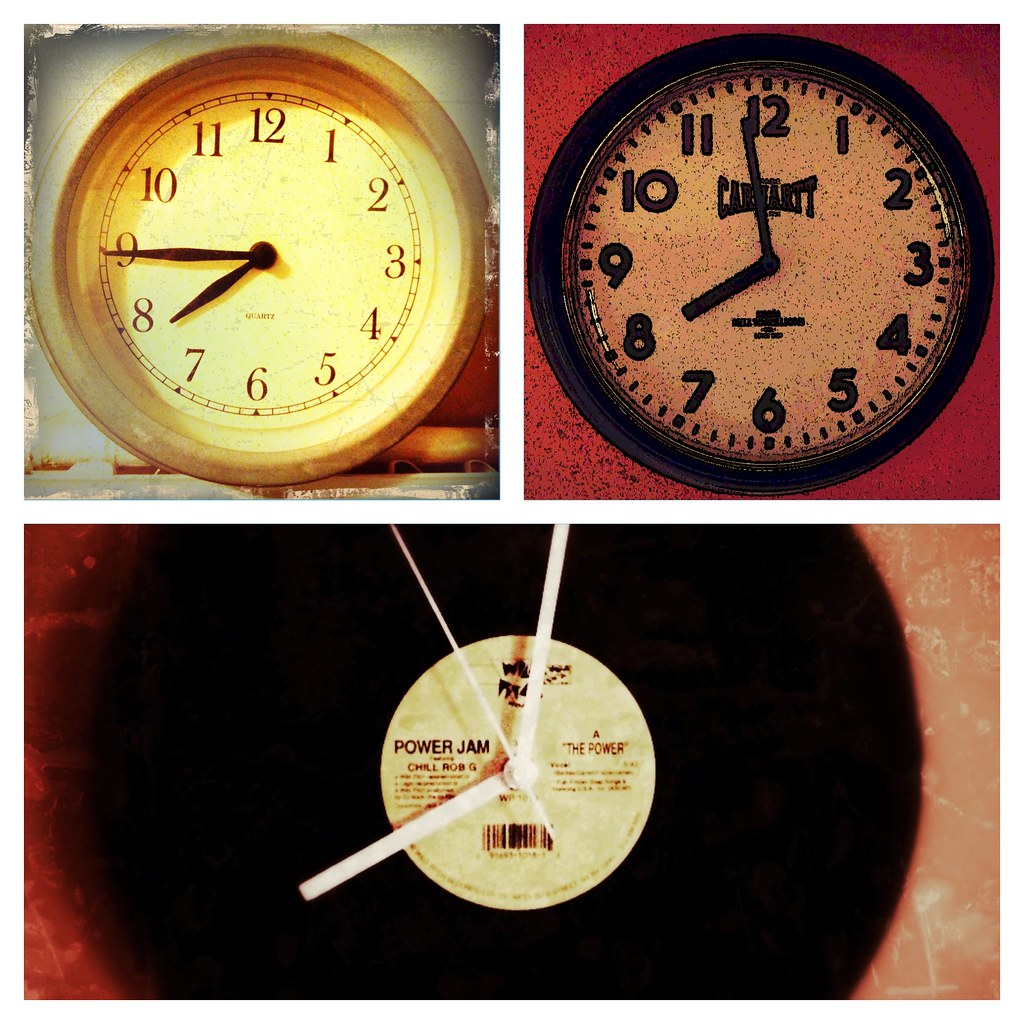The image features three distinct wall-mounted clocks arranged in a triangular pattern, with two at the top and one at the bottom. 

The top left clock has a white face with a subtle tan rim, currently displaying the time as approximately 7:45. 

The top right clock also has a white face but features purple numerals and hands. Due to the dim lighting, details are a bit obscured, but the time appears to be around 8:00. 

The clock at the bottom is uniquely designed to resemble a vinyl record, with no numerals marking the hours. It prominently displays the phrase "Power Jam" at its center. This quirky timepiece also shows the time as roughly 8:00.